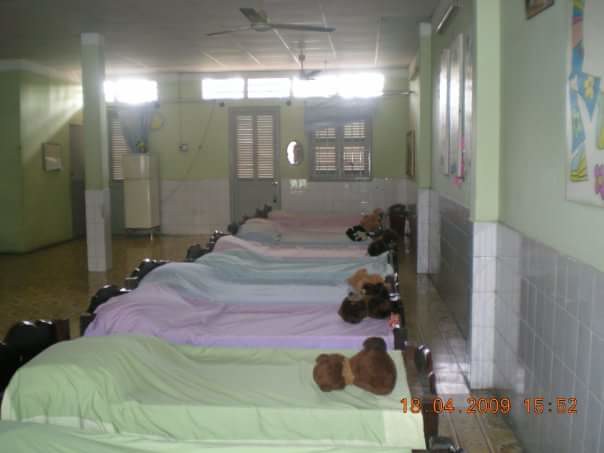In a photo dated April 18th, 2009, a room is depicted with a neat row of small children's beds, each adorned with pastel-colored blankets in shades of pink, blue, purple, and green. The walls of the room are divided with white tiles up to mid-height and painted light green above, crowned with narrow windows near the ceiling. The flooring is a nondescript brown. Each bed, housing a unique plush toy—though the specific types are unclear—contributes to the cozy yet institutional atmosphere. The setting suggests a children's ward or a care facility, underscored by the utilitarian door and window blinds as well as a structural column standing centrally in the room. The photograph captures the essence of a carefully arranged sleeping area designed for children's comfort within a formal setting.